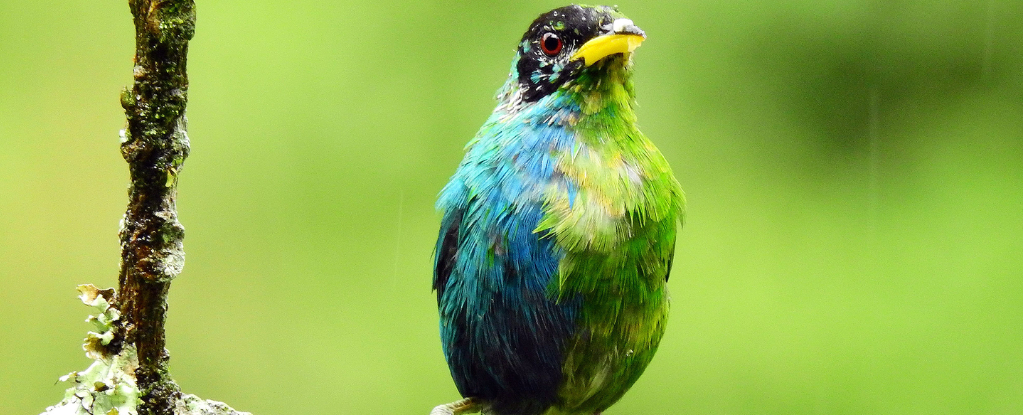This outdoor color photograph prominently features a stunning and colorful bird against a blurred, bright green background with a dark shape in the top right corner. The horizontally long image captures the bird almost at its full height in the center. The bird has a striking appearance with a black head speckled with white or sand-like particles, a single visible red eye looking slightly towards the camera, and a bright yellow beak. Its body coloration is uniquely divided vertically: the left side showcases a vibrant mix of green, yellow, and white, while the right side transitions into an aqua teal hue. A slender vertical branch runs parallel to the bird's body on the left side of the frame, but the bird's feet are not visible in the shot. Despite its textured plumage, the bird's vivid and distinct color pattern stands out clearly against the softly blurred green backdrop.